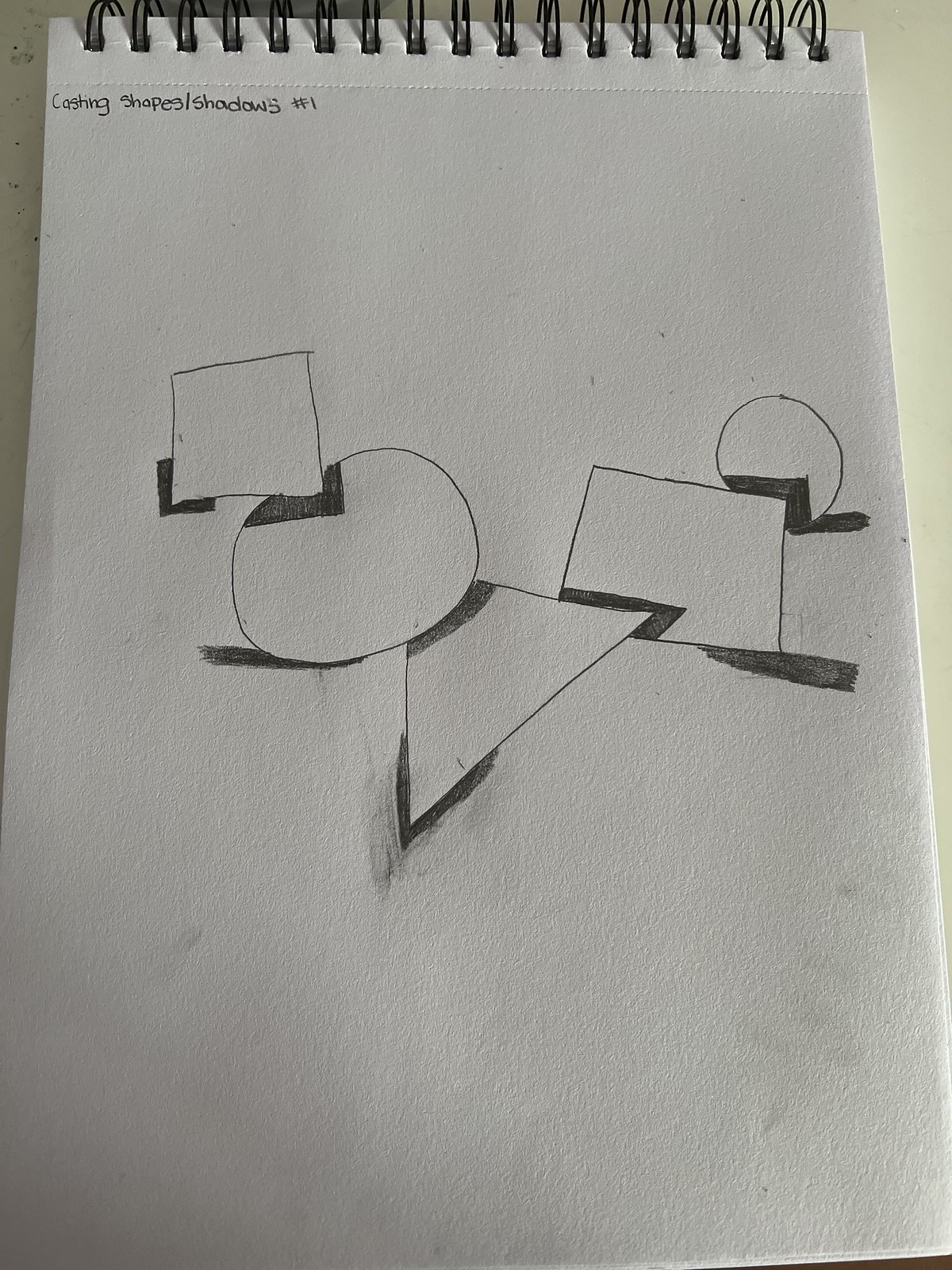The image depicts a detailed drawing on a spiral-bound notepad, with each section featuring double loops for added durability. The spirals, paired in sets of two, run along the entire top edge of the notepad. Directly beneath the perforated line, which allows for easy removal of sheets, the notepad is labeled with the text "Casting Shapes / Shadows, Number 1."

At the heart of the drawing, a sequence of geometric shapes are carefully arranged and intricately shaded to cast realistic shadows. At the top of the arrangement is a square, with its shadow extending below. Connected to this square is a circle, with a shadow where the two shapes meet. The circle then transitions into a triangle, surrounded by shadows that emphasize its form. This triangle links to another square, with the connection point casting further shadows. Above this square, there is another circle, adding to the complexity of the composition.

Each shape and its corresponding shadow are meticulously illustrated, showcasing a study in how three-dimensional forms interact with light and create shadows. The careful attention to detail highlights the spatial relationships between the shapes, resulting in a visually engaging and educational piece.